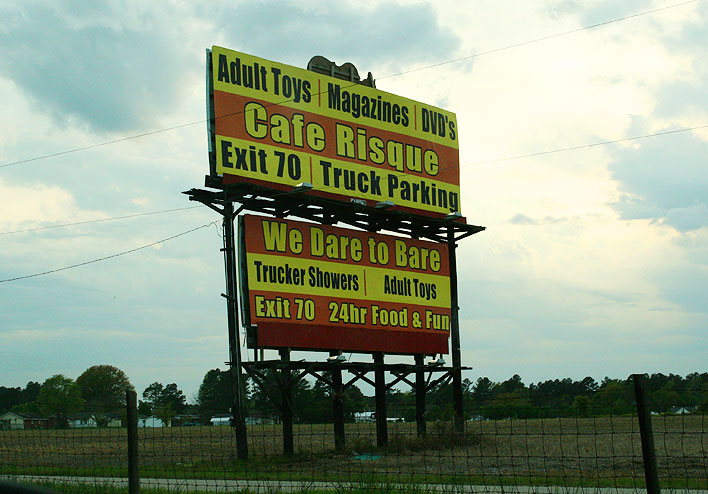The image depicts a large, eye-catching yellow and red billboard in a field alongside a road. The sky above is a vibrant blue with both fluffy white and darker gray clouds, indicating sunlight peeking through. A row of trees lines the upper left to upper right of the image, with electrical cords stretching across the sky. Below, a black metal fence with wooden posts and chain links runs from the bottom left to the bottom right, enclosing a grassy area and separating the field from the road.

The dominant yellow and red billboard features several messages in bold black writing against a yellow background and yellow writing against a red banner. The topmost section advertises "Adult Toys, Magazines, DVDs." Below, a red banner displays "Cafe Risque," followed by another line reading "Exit 70, Truck Parking." The message continues on a secondary billboard below, which boldly states, "We Dare to Bear," and includes additional services such as "Trucker Showers, Adult Toys," and promotes "Exit 70, 24-hour Food and Fun."

In the background, beyond the billboard, there are hints of farm buildings, including a brick house and a white house, and a field with brown, possibly fallow cropland. The overall scene is bright and open, with the natural elements of the sky and landscape contrasting against the vivid commercial signage.